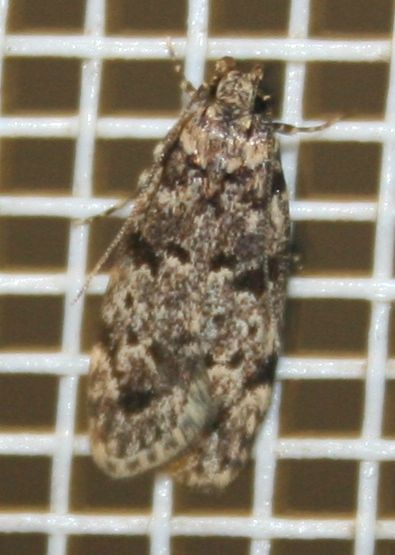In this highly detailed image, a brown mottled moth is resting diagonally on a white grid-like surface, possibly resembling a net or tile, which adds to the intricate composition of the photograph. The image, taken from an overhead perspective, captures the moth in a stationary pose with its wings folded over each other, displaying varying shades of brown and blotches of dark and light patches that suggest it would easily blend into the bark of a tree. The moth's delicate antennae and legs, light mottled in color, are visible, adding finer details to its appearance. The grid beneath it features small squares created by threads running horizontally and vertically. The setting appears to be indoors, with the moth positioned centrally in the image, showcasing its textured environment and the natural elegance of its camouflaged body.